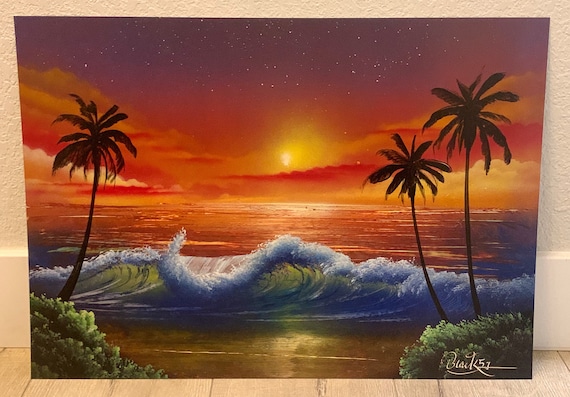This painting, propped up against a white wall on a light wooden floor, captures an ocean front scene at sunset. Dominated by vivid colors, the artwork depicts a large, curled wave in bluish-green hues with a white crest, ready to crash onto the shore. In the foreground, green bushes occupy the lower left and right corners, with a single palm tree on the left and two on the right. The ocean behind the wave is calm and reflects a dark orangish tint from the setting sun. Surrounded by red and yellow clouds, the sun casts a warm glow over the scene, transitioning into a dark purple night sky dotted with small white stars. The interaction of light, colors, and natural elements creates a dynamic yet tranquil coastal vista.